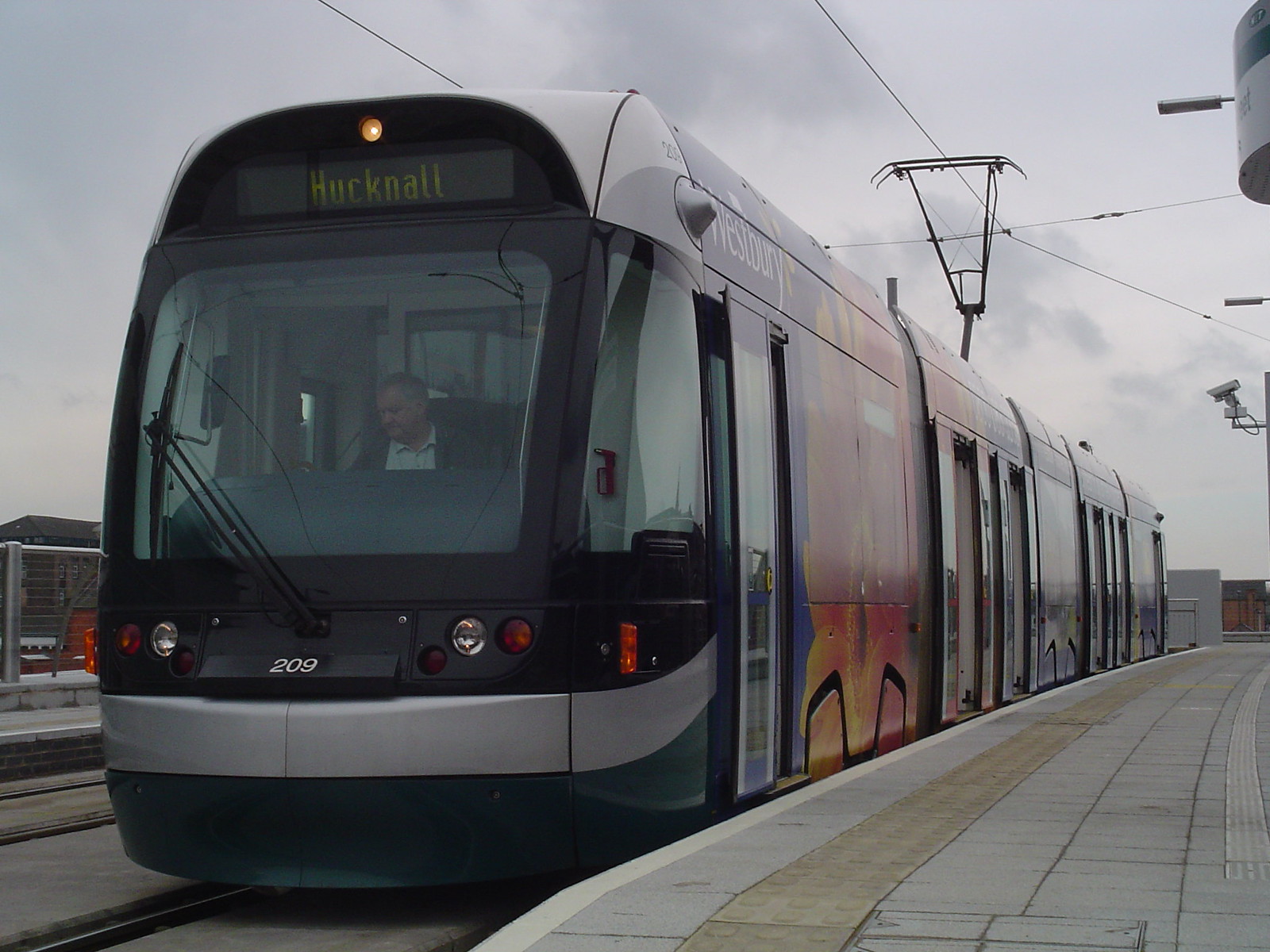This detailed image portrays a commuter train, likely a metro or subway, stationed on its tracks under a gray, cloudy sky. The photograph, taken from an angle showcasing the front left side of the train, reveals the destination "Hucknall" prominently displayed in yellow letters across the top of the train's front. Below the sizable windshield, where an elderly male driver in a light shirt and sweater is visible looking down to his left, the train is marked with the number "2019" (or possibly "209" due to conflicting observations). The front of the train is primarily black with various reflective colors including yellow, blue, and red along its side panels.

The side view extends back, showing multiple compartments with several doors. Orange writing is faintly visible on the front panel, though reflections obscure some details. The ground platform adjacent to the train is made of cement blocks, and train tracks are visible at the bottom left of the image. Overhead, wires can be seen running, likely for power supply, and a security camera is pointed towards the train, maintaining vigilance. The overall lighting suggests the photo was taken near dawn or dusk, contributing to a subdued ambiance of the scene.